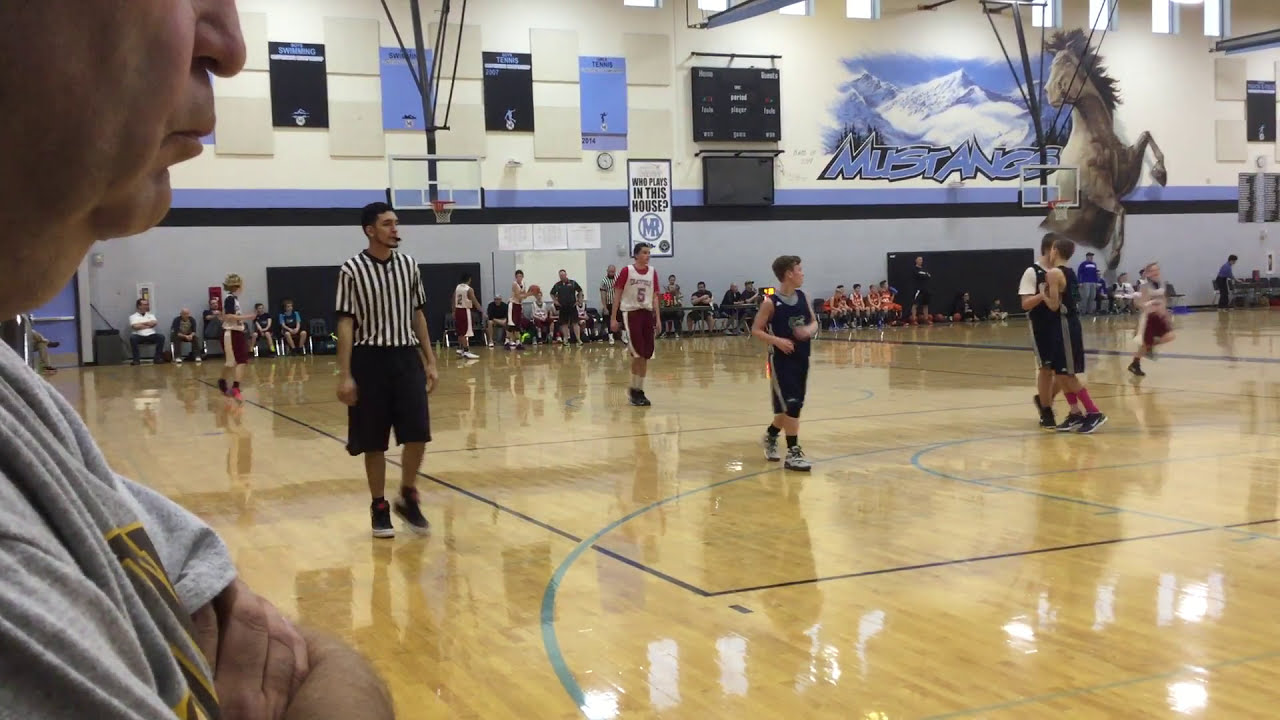The image captures a lively basketball game in what appears to be a junior high or high school gymnasium. At the center of the scene, young boys are actively playing on a highly reflective, glossy court marked with black and green lines and arches. The teams are distinguishable by their uniforms—one in red and white, the other in black. Three boys in dark blue uniforms are positioned to the right side, with one boy in motion, blurred as he runs down the right edge of the court. On the left side, a referee in a black and white striped shirt, black shorts, and a whistle is walking along the sideline.

In the foreground, partially visible is a man in a light gray shirt with his arms folded; only the lower part of his face and his torso are shown. Behind the action on the court, spectators, a mix of boys and adults, are seated along the back wall. This wall is adorned with a mural featuring a prominent illustration of a mustang horse, a snow-capped mountain range, and the word “Mustangs” boldly painted. A black scoreboard is centrally positioned above the mural. Additionally, a rectangular poster reads "Who plays in this house," with a circular logo containing an "M" and an "R." The gymnasium’s high windows let in natural light that, along with the indoor lighting, reflects brightly off the shiny basketball court, enhancing the dynamic and energetic atmosphere of the scene.